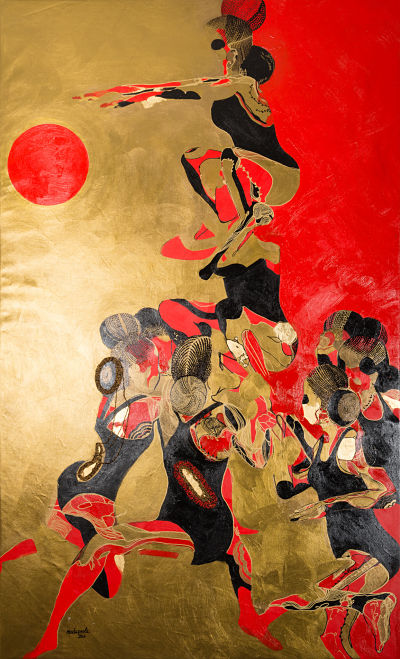The image depicts an abstract, stylized artwork resembling a dance or acrobatic performance. The composition is tall and portrait-sized, with a bifurcated background: the left side is a beige or golden color featuring a prominent red circle near the top, while the right side transitions to a bright red. Central to the artwork is a group of young women, possibly a dance or acrobatic troupe, dressed in black leotards or swimsuits, their hair styled in buns. These women are arranged in a dynamic, multi-layered formation that rises from a busier group at the bottom. One woman stands out in the middle, crouching down on another's shoulders with her arms extended in front of her, suggesting a poised balance or preparatory movement. The juxtaposition of shapes and colors—black, beige, and red—creates an abstract, intriguing depiction of human forms that evoke motion and unity.